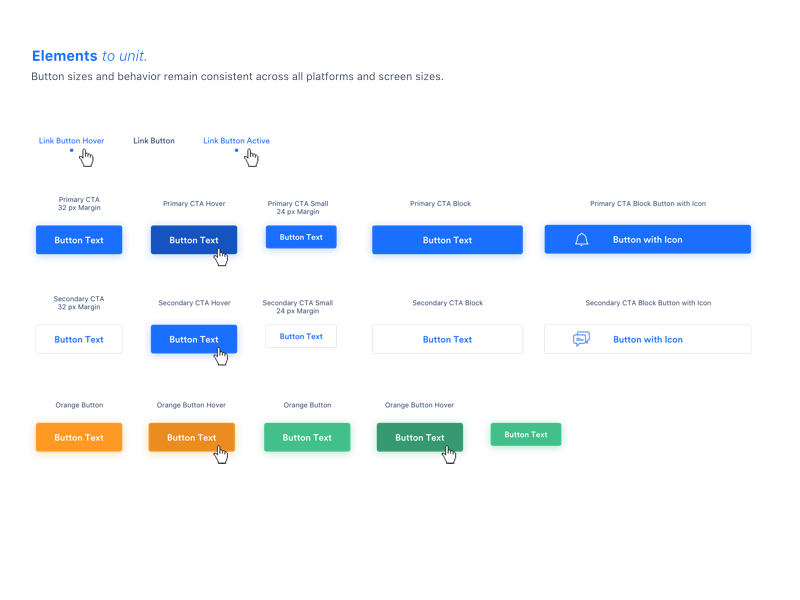The image showcases a detailed layout of a website section titled "Elements to Unit," prominently displayed with a blue heading in the top left corner, where the word "Elements" is in bold. Below the heading, a sentence states, "Button sizes and behavior remain consistent across all platforms and screen sizes."

Following this text are several sections featuring various button styles and states. The first section lists three labels: "Link Button Hover," "Link Button," and "Link Button Active." Both "Link Button Hover" and "Link Button Active" are highlighted in blue with dots underneath them.

Below this, a series of five blue buttons are displayed, each with distinct captions and varying sizes:
1. A medium-sized button labeled "Primary CTA."
2. An identically sized, dark blue button labeled "Primary CTA Hover."
3. A slightly smaller button labeled "Primary CTA Small."
4. A much larger button labeled "Primary CTA Block."
5. The largest button, "Primary CTA Block Button with Icon," which accommodates an icon.

Further down, a row of buttons appears, characterized by a mix of white and blue colors. These buttons maintain similar sizes to the ones above, except the second button is a lighter blue.

The final row consists of five buttons: the first two are orange, and the last three are green. A consistent theme among these buttons is their color behavior when a cursor hovers over them:
- Blue buttons turn a darker shade of blue.
- White buttons turn blue.
- Orange buttons become a darker orange.
- Green buttons change to a darker green.

This visual representation emphasizes the consistency and interaction behavior of buttons across different states and platforms in the user interface.